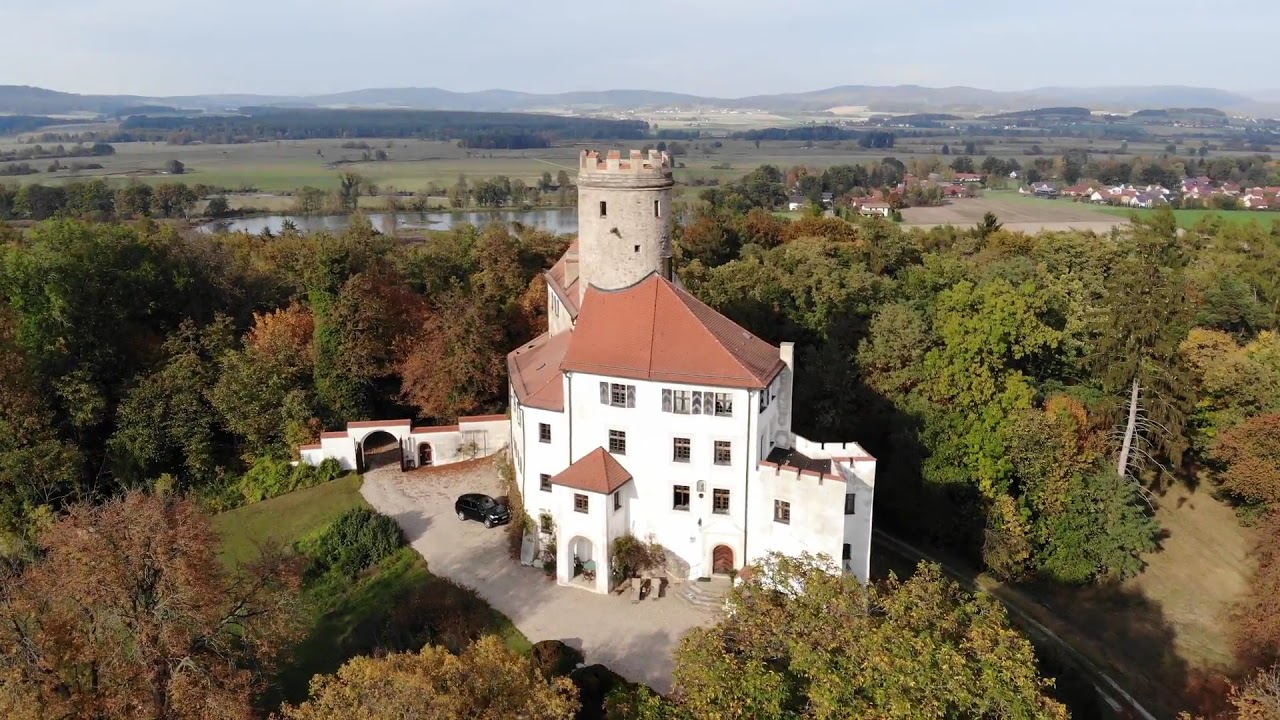The image captures a striking aerial view of a picturesque scene dominated by a prominent light gray stone castle with distinctive architectural features. The castle, with its whitewashed facade and brick-red roof, is centrally positioned on a gently sloping hill, surrounded by lush deciduous and a few evergreen trees. Its most notable feature is a tall, cylindrical tower in the middle, reminiscent of a rook from a chessboard, adorned with small windows that give it a fortified appearance. Below, there's a courtyard where a black SUV is parked, indicating a driveway leading up to the main arched entryway. The scene extends beyond the castle, where rolling green pastures merge into a vivid woodland area, and further back, a serene body of water glistens under a blue-gray sky. To the right, a charming village with smaller houses dots the landscape, all set against a backdrop of modest, snow-free mountain ranges. The trees exhibit a seasonal palette of green, reddish, and orangish hues, hinting at the onset of autumn. The entire scene is bathed in the bright sunlight of a clear day, enhancing the vibrant colors and tranquil beauty of this enchanted location.